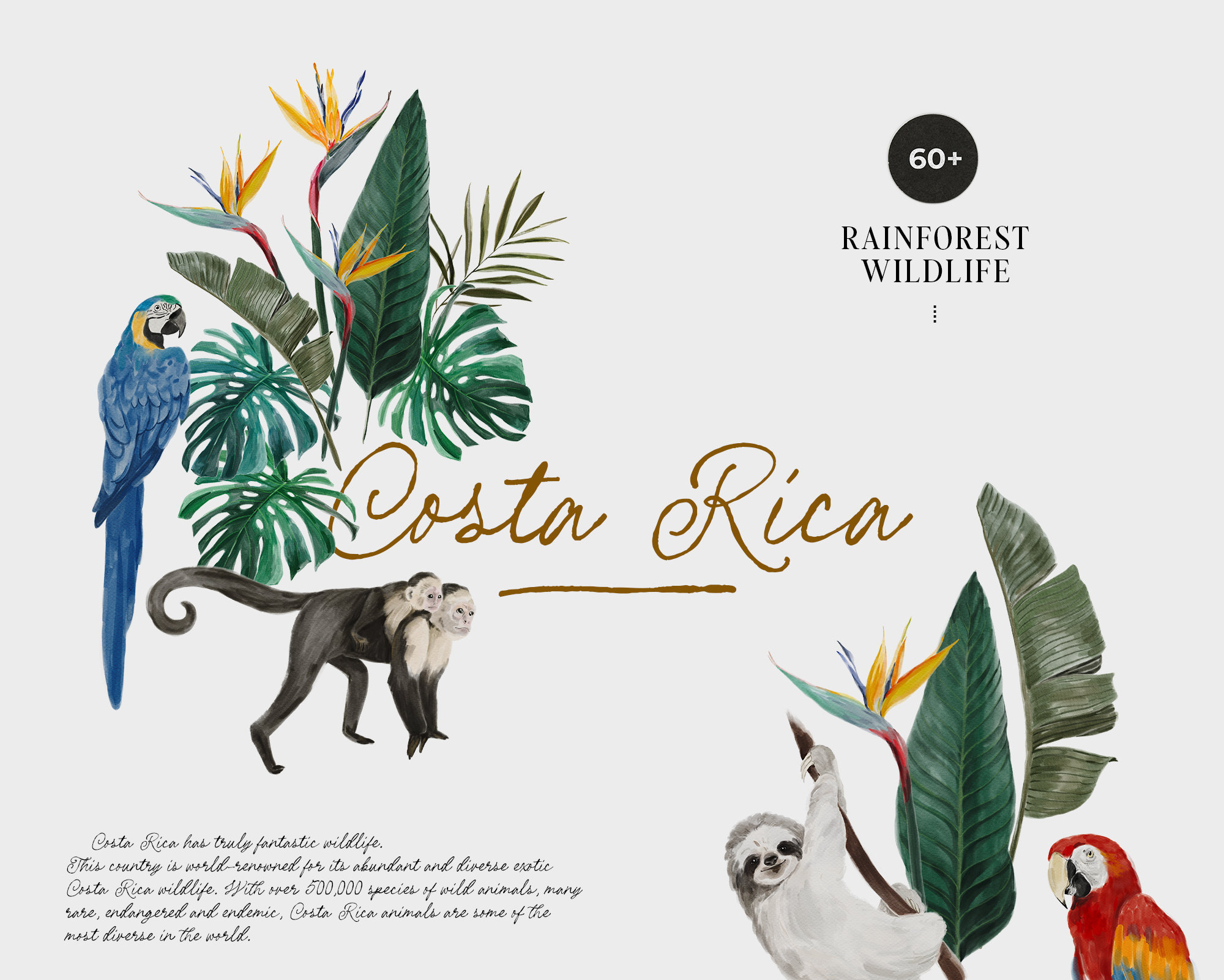This travel brochure for Costa Rica features a beautifully illustrated design on a white background. The top right corner showcases a black circle with white numbers indicating "60 plus," with the words "Rainforest Wildlife" written in black letters beneath. On the left side, tropical foliage, including palm leaves and Birds of Paradise flowers, surround a striking blue Hyacinth Macaw. Centered in flowy, handwritten gold script is the text "Costa Rica,” emphasized by a decorative underline.

Accompanying the lively greenery are two playful monkeys, appearing to be a mother and her baby, conveying a sense of the lush, vibrant wildlife. Towards the bottom right, a light-colored three-toed sloth hangs from a tree branch amidst more tropical leaves and flowers. Nearby, a brilliantly colored Scarlet Macaw, with its red, yellow, blue, white, and black plumage, adds to the vivid scene.

Below the main elements, on the left-hand side in elegant cursive script, there is text detailing Costa Rica's rich biodiversity, though it is largely unreadable. The main focus of the caption emphasizes the nation's reputation for its abundant and diverse wildlife, featuring over 500,000 species, many of which are rare and endemic.